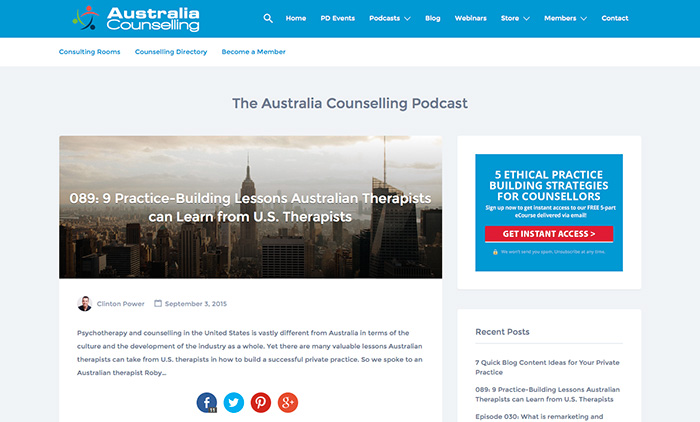This image is of the homepage of the website "Australia Counselling." The site features a variety of dropdown menus and search functionality prominently displayed at the top. Menu options include "Home," "PD Events," "Podcast," "Blog," "Webinars," "Store," "Members," and "Contact." Below these are sections labeled "Consulting Rooms," "Counselling Directory," and "Become a Member." 

The central section of the homepage displays an image likely depicting a city skyline in Australia with several tall buildings under a slightly hazy sky. The page also features a headline reading "089: Practice-Building Lessons Australian Therapists Can Learn from US Therapists," contributed by Clinton Power on September 3, 2015. Below the headline, there is a brief introductory paragraph on psychotherapy.

On the right side of the page, a highlighted box titled "Five Ethical Practice-Building Strategies for Counselors" offers instant access to resources, with the call-to-action "Get Instant Access" prominently displayed in red. Additionally, the webpage includes a section for recent blog posts.